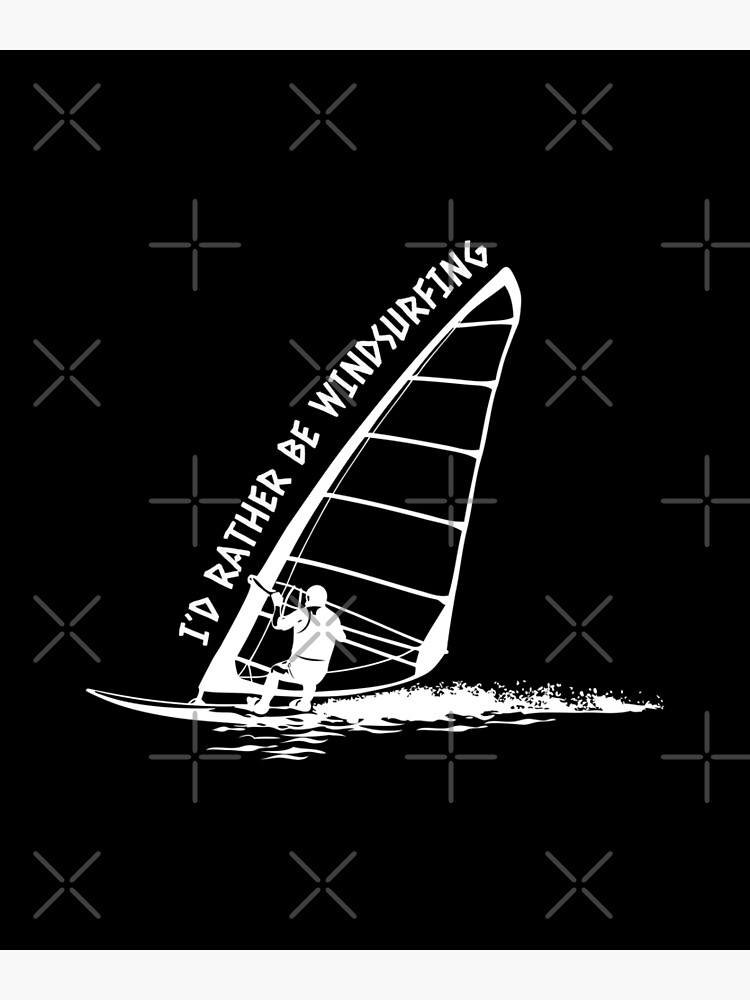In this image, we have a striking illustration set against a black background, featuring a dynamic white silhouette. Dominating the scene is a tall sail, around which the phrase "I'D RATHER BE WINDSURFING" is boldly displayed in capital letters, seamlessly following the shape of the sail. A figure, clad in a white outfit complete with a helmet and gloves, is depicted windsurfing, gripping a rope that wraps around the sail. The person appears to be moving towards the left side of the image, with water foaming up behind them, indicating motion and speed. The background is further accentuated by a repeating pattern of gray X's and crosses, adding texture and depth to the composition.